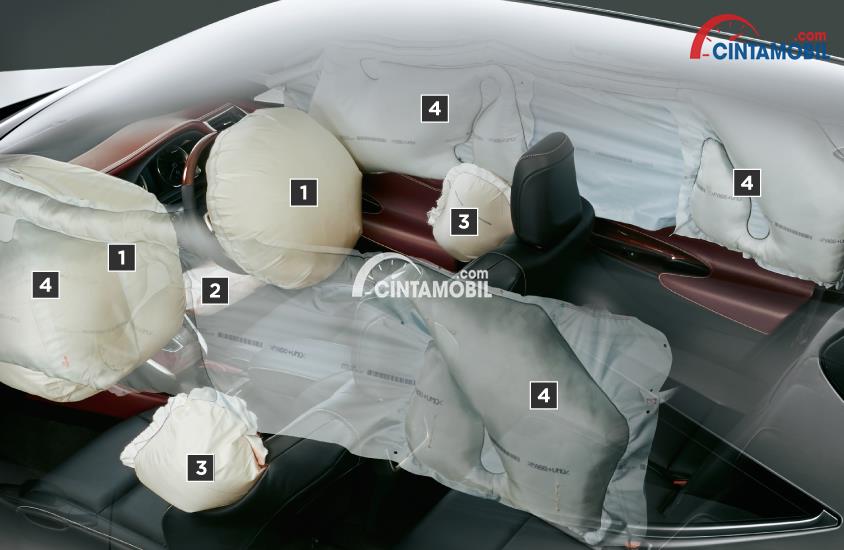The image depicts the interior of a vehicle, potentially a sedan or SUV, with a prominent watermark reading "sentomobile.com" at its center, indicating it is a mobile vehicle. The car features black leather seats and red leather trim on the doors and the dashboard. The steering wheel, located towards the left side of the image, is partially wooden and brown. The vehicle's interior is confusing to interpret at first due to multiple airbags being deployed – an airbag in the steering wheel, additional airbags on the side of the headrest and seats, and a large airbag covering the side of the car. The cloth covering seen over many car components initially hinted at damage or a special condition. This cutout or graphic of the car also includes various numbers in gray squares with white lettering that designate each airbag. The image's details suggest a visualization for airbag deployment within the vehicle. In the top-right corner, the provider name "sintemon.com" is displayed in red and blue lettering.